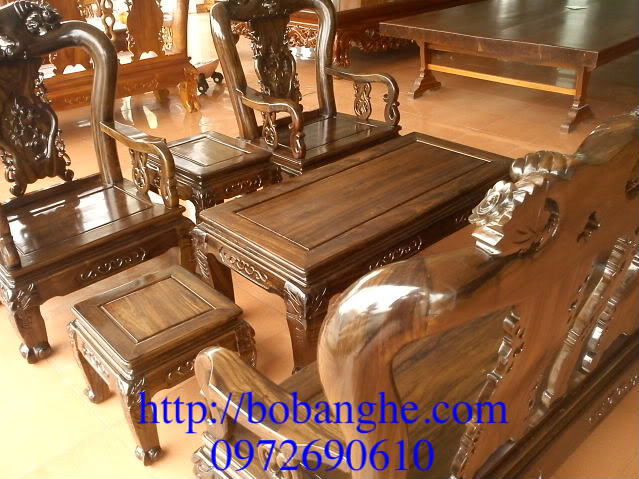This photograph depicts an elegantly furnished interior, likely a showroom, showcasing elaborate wooden furniture. Dominating the scene are two ornately carved dark wooden armchairs, reminiscent of thrones, with intricate scrollwork and paw-shaped legs. Between them sits a similarly carved small table. In the foreground, there is a matching coffee table and a small side table, while the back of a carved wooden loveseat or bench is also visible. All the furniture features a shiny finish, emphasizing its antique, possibly Victorian or French Provincial style. The setting is complemented by a light orange or salmon-colored shiny tile floor. The background reveals an array of additional carved wooden pieces, suggesting that the space is filled with high-end furniture. Superimposed in blue at the bottom of the photograph is the text "http://bobanghe.com" followed by the number "0972690610," indicating the furniture is for sale.